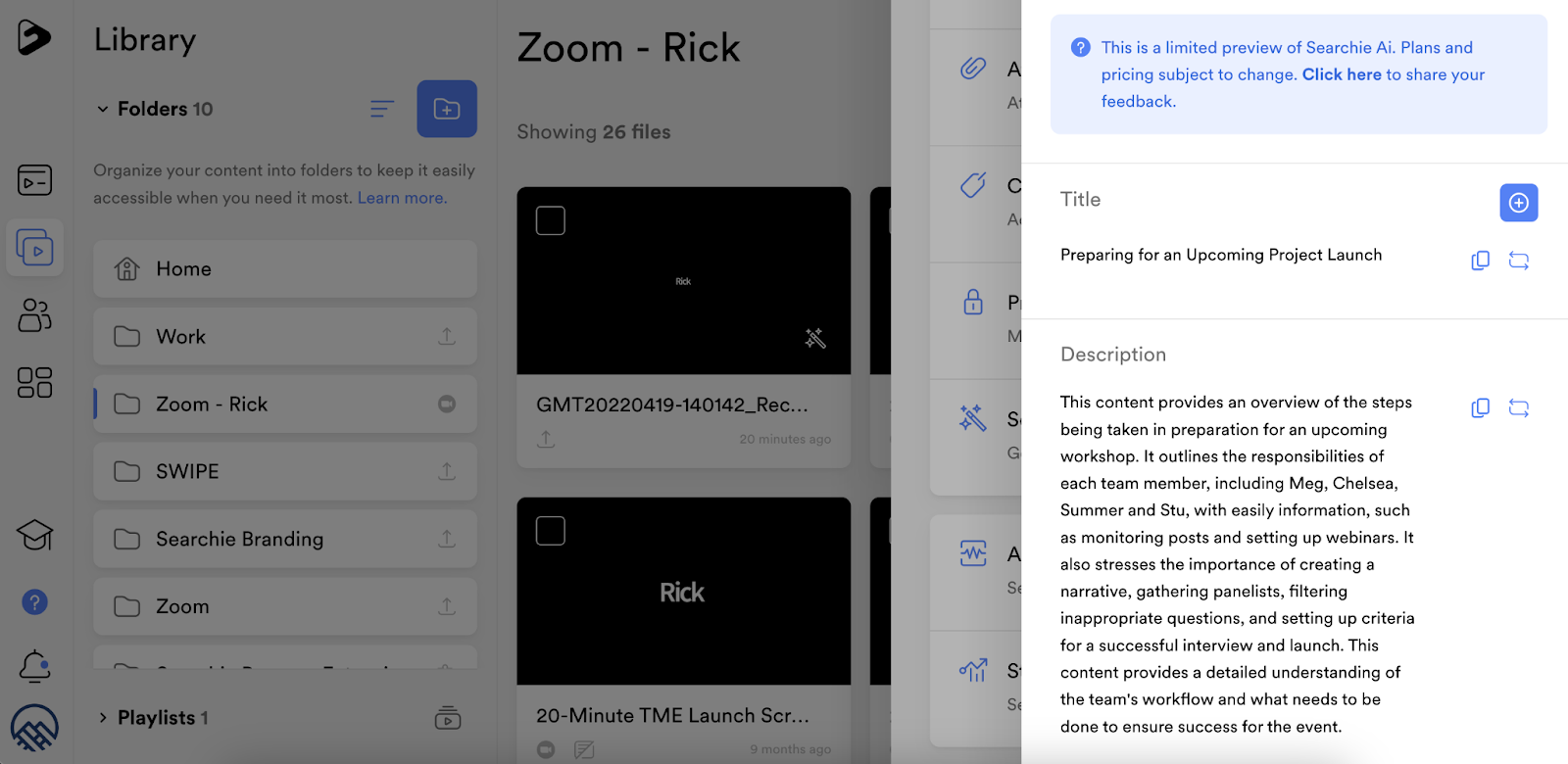This screenshot captures the dashboard of a website or app with a user interface designed for navigation and management. The right side of the screen is tinted dark, showcasing a section titled "Library" at the top left. Directly below this title, there is a dropdown menu labeled "Folders 10," indicating the availability of ten folders. Adjacent to this dropdown is a blue folder icon button.

On the left side of the screen, there is a vertical sidebar featuring several icon buttons. The sidebar includes icons labeled "Videos" and "Profile," as well as an icon resembling a graduation cap, a question mark, an "More Info" item, and a notification bell.

Adjacent to the sidebar on the right are multiple buttons and rectangular-shaped buttons labeled "Homework," "Zoom Rick," "Swipe," "Searchie Branding," and "Zoom."

At the top of the right section, there is a blue information box containing the text, "This is a limited preview of Searchie AI. Plans and pricing subject to change, click here to share your feedback." Next to this information box, there is a blue plus icon button.

The interface appears highly organized, facilitating easy navigation and providing various functionalities at a glance.